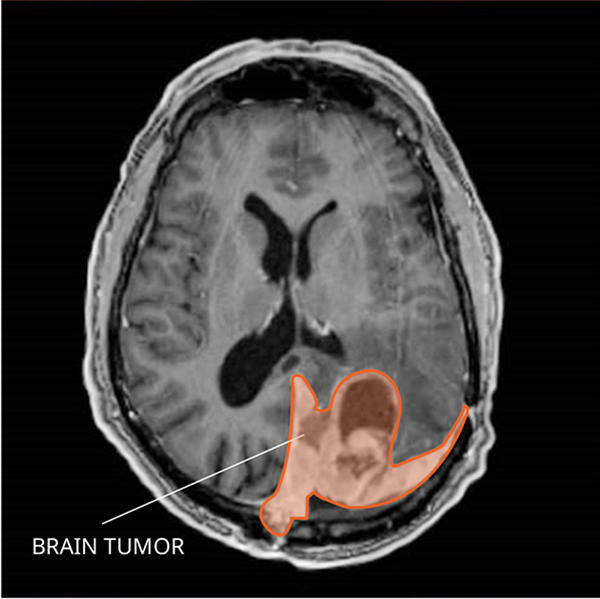In this detailed cross-section image of a human brain, predominantly rendered in shades of gray and black on a stark black background, several distinct features can be observed. The brain itself is mostly gray, with the edges displaying some black areas. The middle of the brain has irregular dark shapes and dense, pitch-black spots towards the center, indicative of natural brain structures. The outer portions and the surrounding skull appear in lighter gray and almost white tones, with the characteristic cauliflower-like curls marking the brain's surface.

Notably, in the lower right corner of the brain, there is a highlighted region marked as a brain tumor. This area is distinctly outlined in dark red or thick orange, with a lighter orange or red fill, making it stand out prominently against the grayscale backdrop. A white label outside of the scan explicitly identifies this area as "brain tumor," with an arrow pointing to the marked region. This comprehensive and detailed imaging presents a clear picture for medical evaluation, illustrating the areas of interest with precision and clarity on a black, X-ray or MRI-like background.